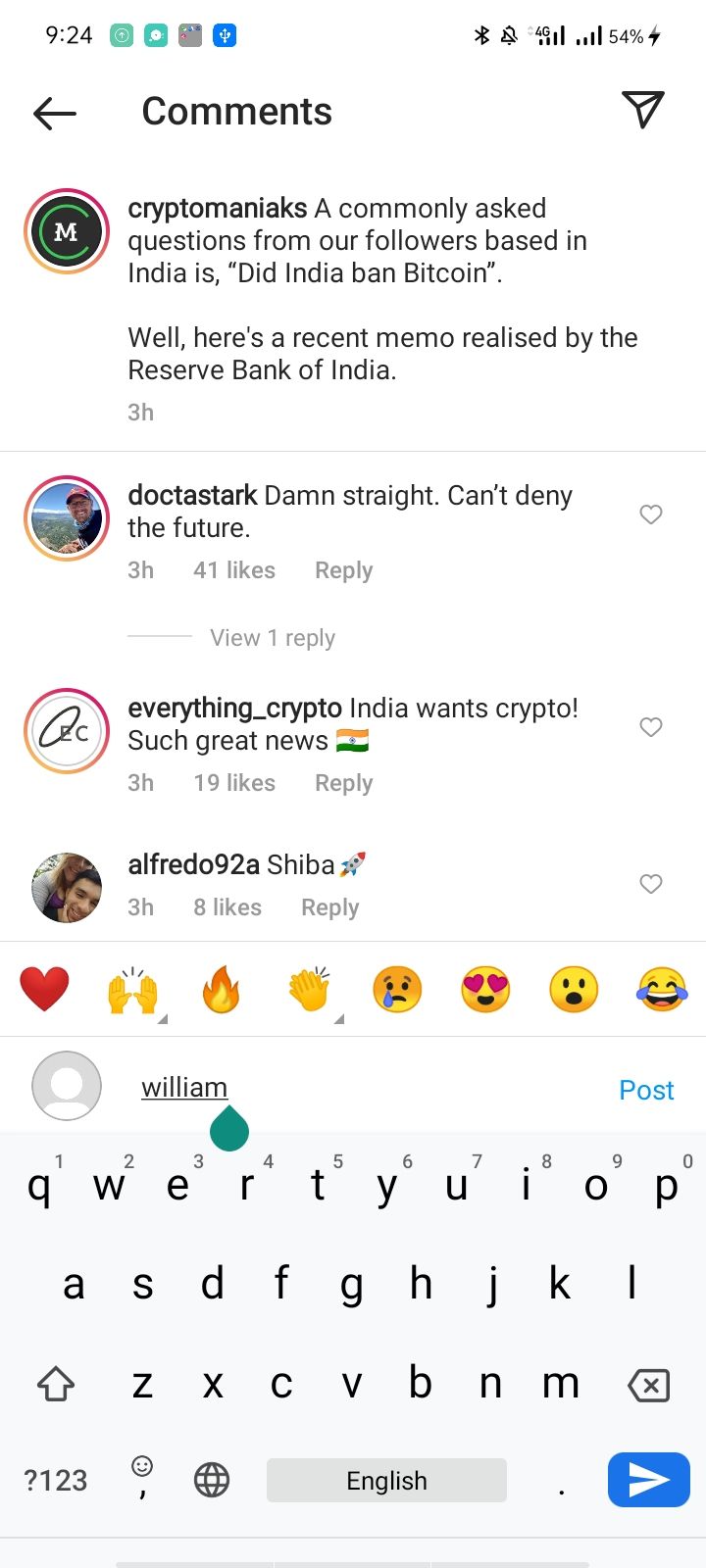This image, evidently a screenshot taken from a mobile device, prominently features a social media comment section along with the typical device status indicators. At the top of the screen, the time reads 9:24, accompanied by four icons. In the upper right corner, there are symbols for Bluetooth, ringer status, and battery percentages.

Directly beneath this, a comment section is displayed. On the left, an arrow points to the word "comments." Adjacent to this is a right-facing triangular arrow, likely indicating additional options.

The comments begin with a circular avatar resembling a profile picture, akin to what one might select on Facebook. The username "Crypto Maniacs" heads the first comment, which addresses a common question from followers in India about the country's stance on Bitcoin. It states: "A commonly asked question from our followers based in India is, did India ban Bitcoin? Well, here is a recent memo released by the Reserve Bank of India." This comment was posted 3 hours ago.

Following this is a line separating another profile comment. The next profile features a man's avatar with the username "Dr. Stark," who comments, "Damn straight, can't deny the future," also posted 3 hours ago. This comment has received 41 likes and an option to reply with a note that there is one existing reply, not visible due to the screenshot.

Subsequently, the profile "everything_crypto" comments, "India wants crypto! Such great news," with an accompanying Indian flag emoji. This comment also posted 3 hours ago, has garnered 19 likes. 

The user "alfredo928," with a profile name "Sheba" and a rocket icon, posted another comment 3 hours ago, achieving 8 likes.

Below "alfredo928" is a line separating various emoji reactions: heart, raised hands, fire, clapping hands, a frowning face, a heart-eyes face, an astonished face, and a laughing-crying face.

The final profile lacks a personalized picture, using a default avatar indicating a male figure. The username "William" is displayed with an underscore below it, suggesting an ongoing input. Below, there is a QWERTY keyboard interface for typing messages, with a blue "post" link to submit the comment once typed.